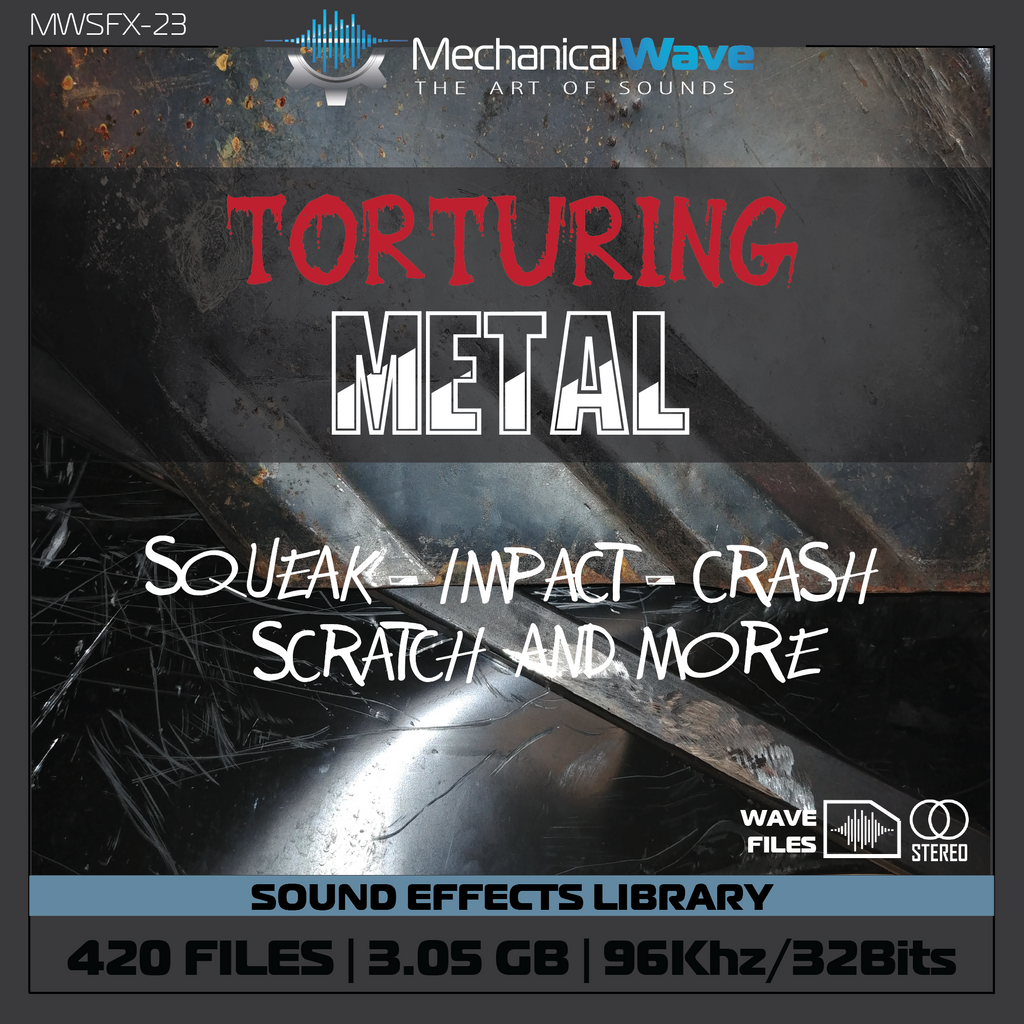The design is a striking album cover with a dark, multifaceted black background featuring a subtle metallic texture. Centered at the top, the title "Mechanical Wave: The Art of Sounds" is prominently displayed, with "Wave" in vivid blue. To the left, a logo with blue sound waves of varying frequencies adds a dynamic touch. Directly below, in dripping red text that resembles blood, the word "Torturing" stands out ominously. Beneath it, the word "Metal" appears with its letters partially cut off at different angles, transitioning from gray at the top to white at the bottom.

Midway down the page, descriptive sound effect words "squeak, impact, crash, scratch, and more" are listed in white text. At the bottom, the technical details of the sound effects library are provided. In white text, it states the library includes "420 files, 3.05 GB, 96 kHz, 32 bits" next to a smaller version of the sound wave logo and an interlinking circle symbol labeled "stereo." Below this information, a blue strip with black text reads "sound effects library," all framed within a dark charcoal gray border.